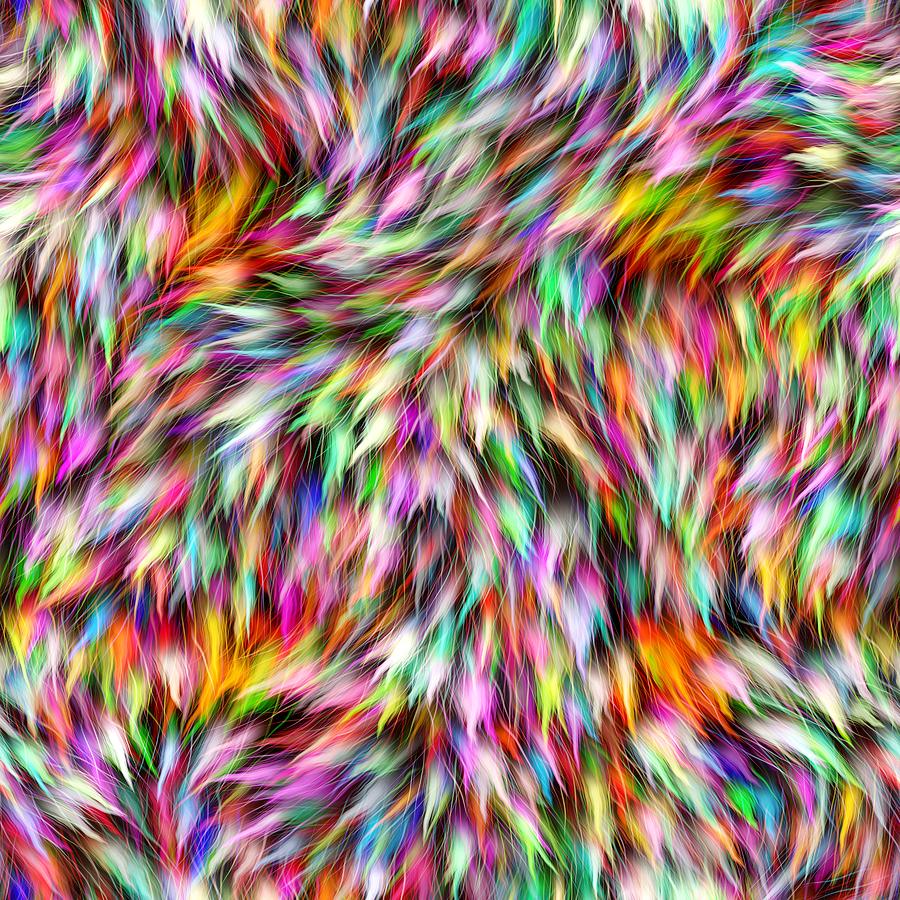The image features a highly intricate and vibrant display that resembles a close-up view of shaggy fur, potentially from a fur coat or a funky rug. The fur strands are vividly colored, almost as if they were tie-dyed, with a spectrum of hues including pink, dark pink, yellow, green, teal, blue, light blue, orange, purple, and white. The colors blend together without any discernible pattern, creating an effect that might even suggest a computer-generated image. This detailed, rainbow-like fur showcases varying lengths, giving an impression of depth and texture, akin to the look of faux fur or an elaborate carpet.